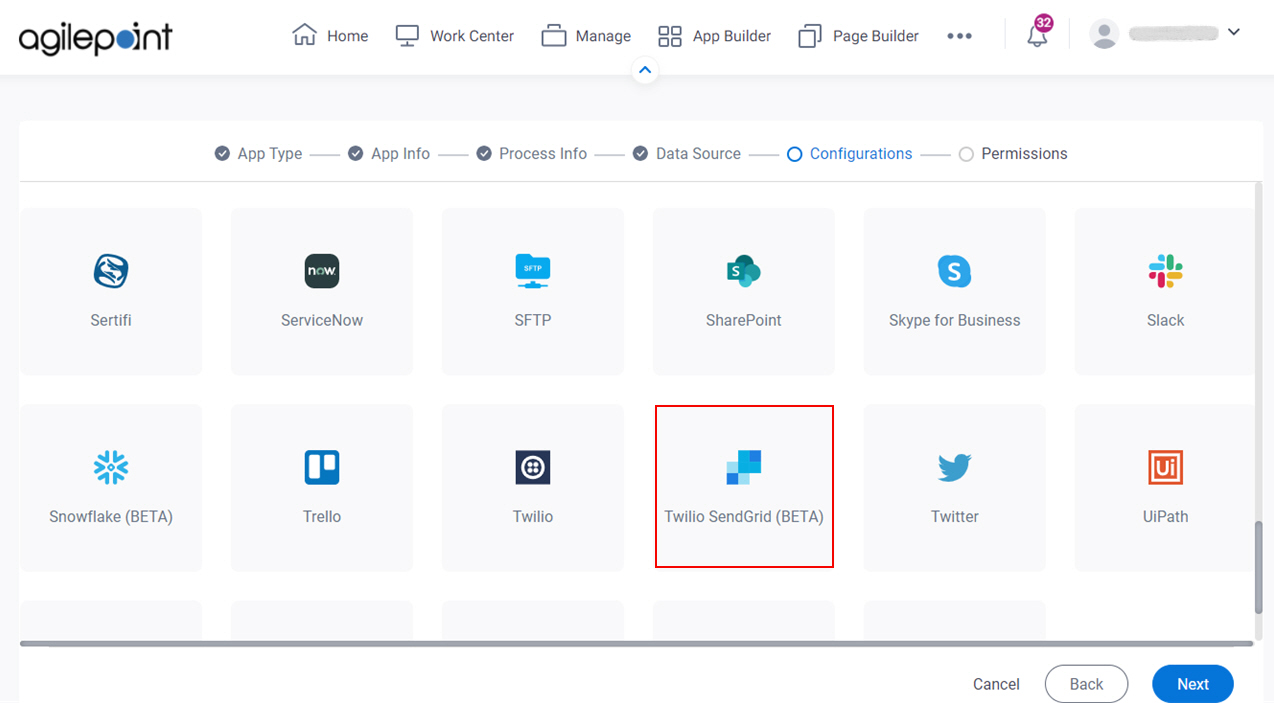The top left corner of the image features the text "AgilePoint," written in black. The 'O' in "Point" is uniquely designed as a blue-shaded circle. At the top of the interface, several tabs are displayed: Home, Work Center, Manage, App Builder, Page Builder, alongside a notification icon and a profile icon. The notification icon is represented by a purple circle, while the user profile icon is greyed out, indicating it is currently hidden or inactive.

Below these primary tabs, a secondary row of tabs is visible, listing: App Type, App Info, Process Info, Data Source, Configuration, and Permissions. The "Configuration" tab is highlighted in blue, indicating it is the current active section, with the previous stages (App Type, App Info, Process Info, Data Source) marked as completed.

Within the Configuration tab, a variety of integration options are presented. From left to right, these options include: CTV, ServiceNow, SFTP, SharePoint, Skype for Business, Slack, Snowflake (Beta), Trello, Twilio, Twilio SendGrid (Beta, outlined in red), Twitter, and UiPath. Some additional options at the bottom are mentioned but not visible in the image.

In the bottom right corner, there are three navigation buttons: a blue "Next" button, a white "Back" button with black text, and one additional button whose details are obscured in the image.